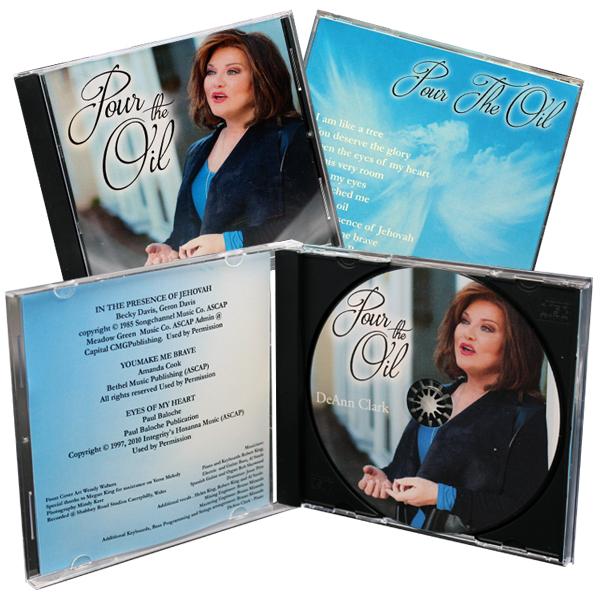The image presents a detailed product display of a CD titled "Pour the Oil." At the top left, you can see the front cover of the CD package, featuring a woman with short, dark hair, possibly in her 50s, wearing a black jacket over a blue shirt. The title "Pour the Oil" is written in cursive dark font to the left of her. To the right, there's another image showing the back cover of the CD, which is light blue with white clouds forming an angelic shape. The back cover also lists the song titles in white.

At the bottom, the CD is shown standing open, displaying both the inside and the CD itself. On the left side of the open package, a blue information sheet lists detailed track information and credits, though the small black font makes it challenging to read. The CD on the right side mirrors the front cover image, featuring the same portrait of the singer and the title "Pour the Oil," along with the name "Deanne Clark" prominently displayed. The background of the display is white, framing the CD and its packaging elements neatly.